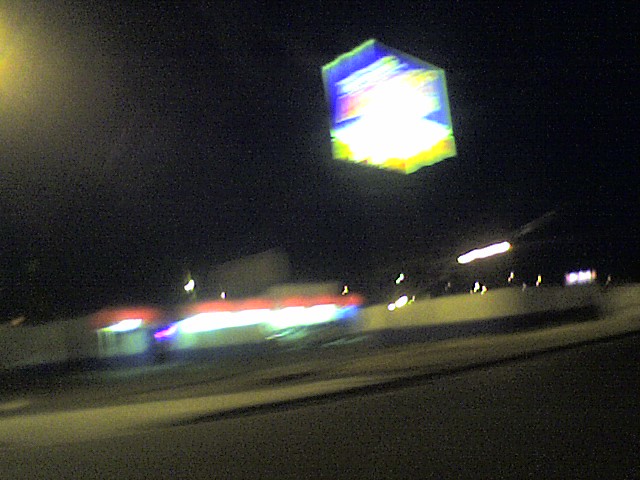The image captures an extremely out-of-focus, nighttime scene looking down a side street. Dominating the hazy view is a highly illuminated sign or billboard suspended in the air, though its structure remains indiscernible. The sign emits a mix of bright blue, white, yellow, and a hint of red, possibly the beginning of a word. In the background, there is a vaguely visible building with lights glowing, including red and white lights which might be part of an awning. The sky is dark, further emphasizing the dimly lit surroundings. Additional scattered lights from other buildings punctuate the distant nightscape. The lower portion of the image shows a gray road beneath the scene, though all details remain obscured by the heavy blurriness.